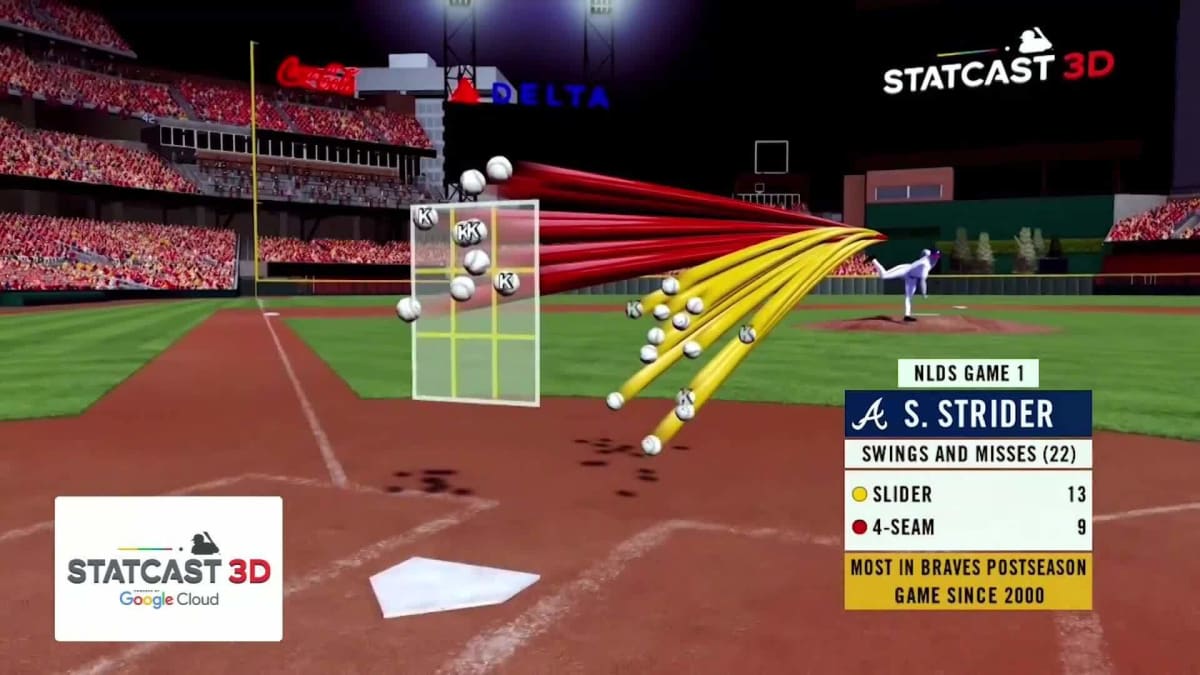In this highly detailed video game screenshot, we are immersed in a vibrant baseball stadium scene, specifically focusing on a pitcher named A.S. Strider standing on the brown muddy pitcher's mound, surrounded by lush green grass. The scene highlights Strider's intense pitching action, with at least 20 baseballs visibly streaking towards their targets; yellow streaks denote sliders with the number 13, while red streaks represent four-seam fastballs, tagged with the number 9. At the bottom left of the screen, the caption reads "A.S. Strider," followed by "swings and misses," "Slider," "Four Seam," and "Most in Braves postseason games since 2000," emphasizing Strider's significant contribution. The bottom right corner features the StatCast 3D Google Cloud logo. Surrounding the field, the stands are filled with an excited crowd, sitting beneath a prominently lit Coca-Cola sign above the bleachers, enhancing the authentic ballpark atmosphere.